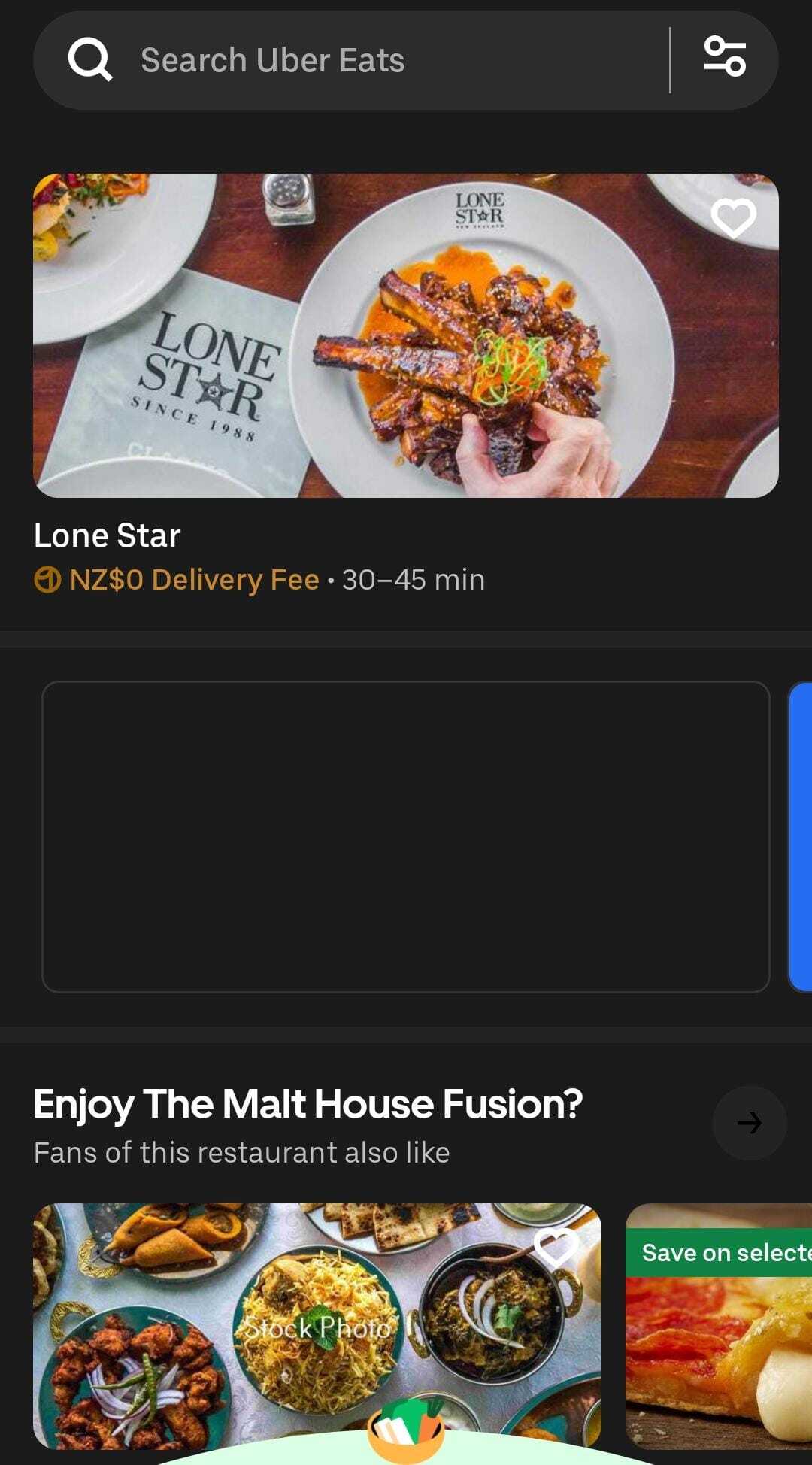The image features a sleek black background with a rounded search bar at the top, slightly lighter in color. The search bar, which includes a white magnifying glass icon, displays the text "Search Uber Eats," with "U," "E," and "S" capitalized.

Beneath the search bar is a detailed graphic depicting a restaurant scene. Central to this graphic are three plates of food, arranged with one plate in the center and two on the sides. A napkin in the graphic bears the inscription "Lone Star Since 1988." A person's right hand, positioned to the left, is seen reaching for food from the plate in front of them.

Text within the graphic reads, "Lone Star, NZ, $0 delivery fee, 30 to 45 minutes," followed by a blank black square. Below this square, text asks, "Enjoy the Malt House Fusion?" with specific letters capitalized for emphasis: "E" in Enjoy, "T" in The, "M" in Malt, "H" in House, and "F" in Fusion.

The bottom section of the image lists "Fans of this restaurant also like," accompanied by various food images labeled "stock photo." Each of these images features a heart icon in the corner, suggesting a favorites or like function.